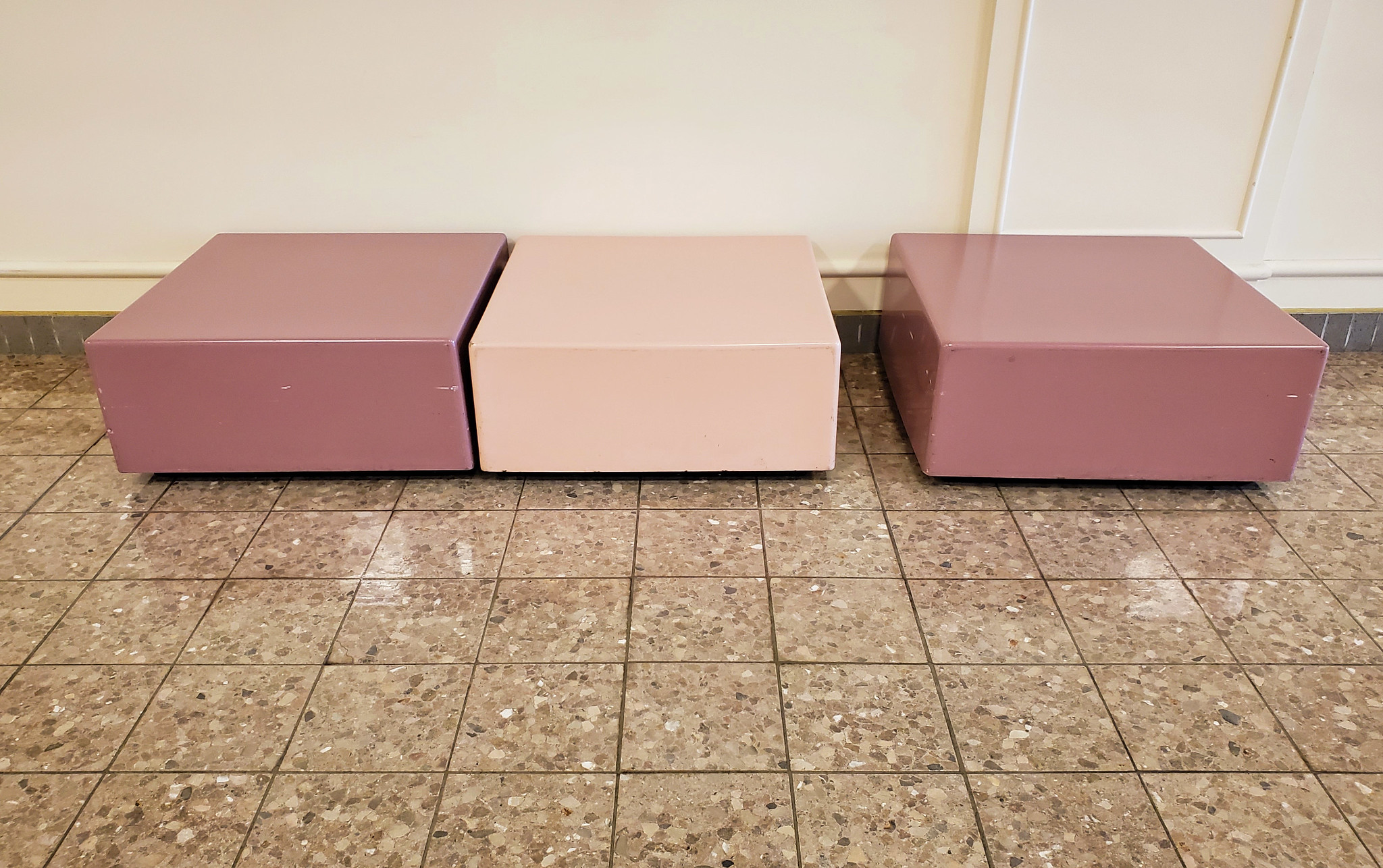The photograph captures three rectangular-shaped seating blocks arranged horizontally on a textured tile floor featuring a mix of browns, grays, and whites. The seating blocks vary in color; the one on the left and the one on the right are a dark cherry or mauve color, while the center block is a lighter peach or creamish beige. Each block appears to be about one and a half to two feet tall, making them suitable for sitting or possibly for step exercises. The arrangement shows the tops and fronts of the left and center blocks, while the right block also reveals its left side. The wall behind them is a tan or cream-white shade, complemented by a distinct molding in a tan color with a brown edge along the bottom. The setting suggests versatility in their use, possibly in an exercise area, a play space, or casual seating in a communal environment.